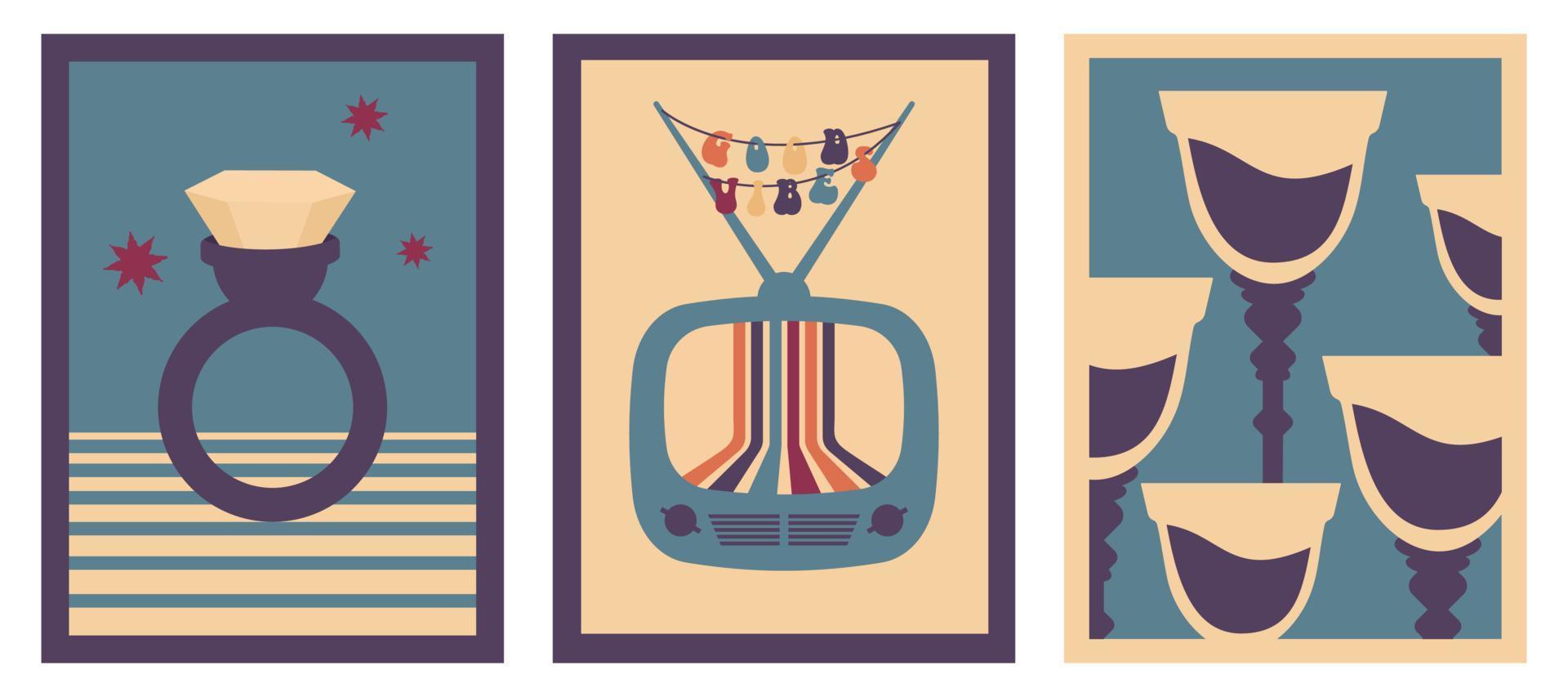The image consists of three digitally created panels arranged horizontally, each framed with distinct borders. The left panel, bordered in navy blue, features an illustrative depiction of a ring with a navy band and a large, white, cartoon-like stone adorned with red stars against a light blue background. Below the ring, beige stripes add subtle detail. The central panel, bordered similarly in navy blue, displays a retro teal blue television with antennas. The TV screen shows curved, multicolored vertical stripes, reminiscent of an old-timey broadcast, with the word "Good Vibes" strung between the antennas. The rightmost panel, with an off-white border, presents five navy blue-stemmed wine goblets, each filled halfway with navy blue liquid, giving an elegant contrast against the panel's minimalistic backdrop. The entire composition incorporates colors such as cream, maroon, orange, yellow, and off-white, creating a cohesive yet vibrant visual symphony.